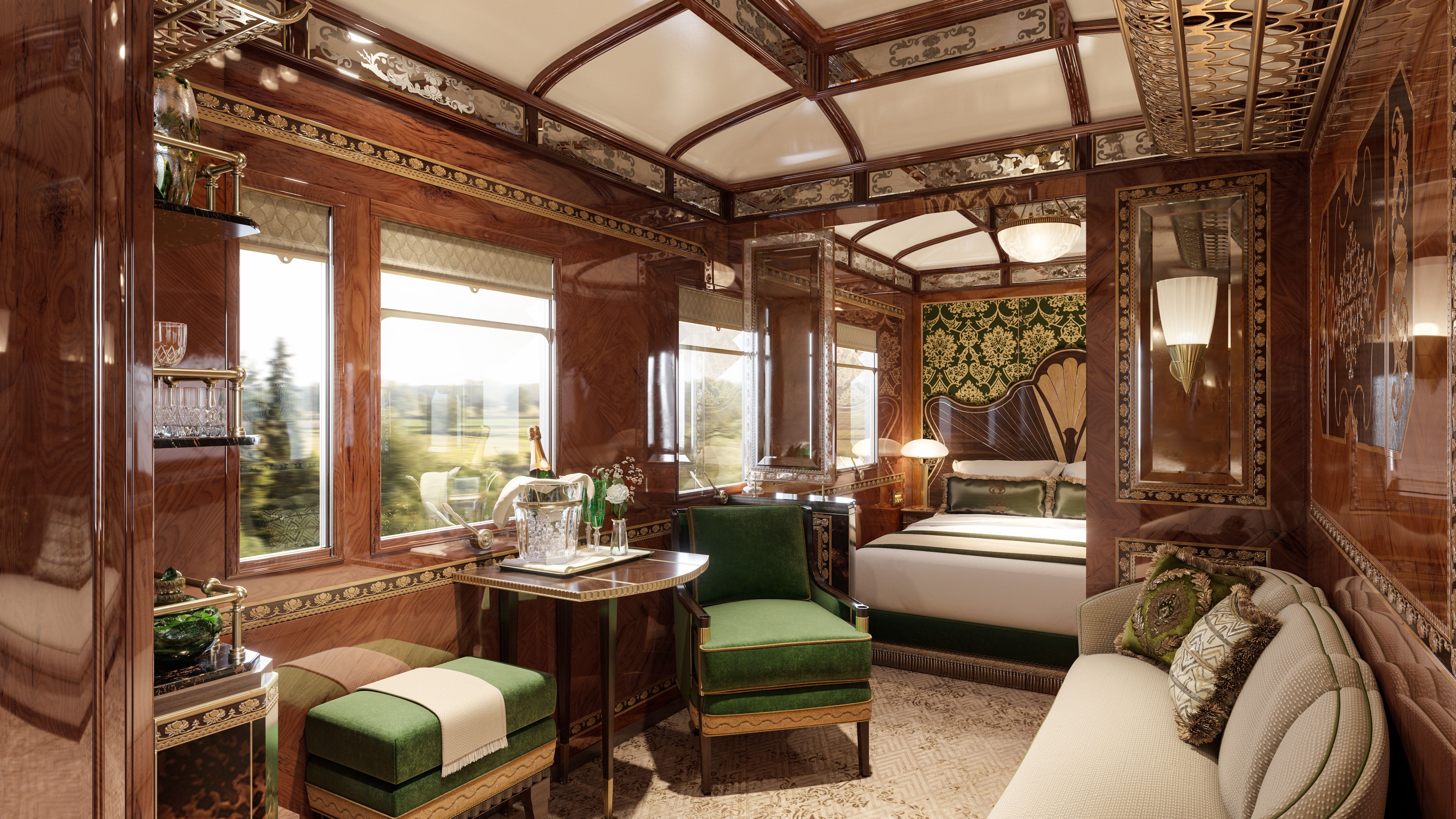The image depicts the inside of a luxurious train car, specifically designed to combine the coziness of a bedroom and a living room. The compartment exudes elegance with its rich wood grain that covers the walls and various pieces of furniture. The setting unmistakably suggests a train in motion, evident from the slightly blurry greenery visible through the four wide windows, which enhances the sense of speed and movement.

At the bottom right corner, there is a beige couch adorned with two pillows, positioned against the wall. To the left of the couch is a chair with green cushions and a brown wooden frame, complemented by a matching stool nearby. Next to the chair, a table holds a bucket of champagne along with glasses, signifying the opulent nature of the space. Further left, a set of shelves display more glasses and additional decorative items, contributing to the luxurious ambiance.

The bedroom area features a pristine white bed with a subtle black border on the bedspread. Decorative pillows sit atop the bed, adding intricate designs to the overall look. Behind the bed, a floral pattern in green and tan harmonizes with a central fan design, all surrounded by the consistent wooden decor. The wood paneling is sleek and polished, which enhances the lavish feel of the train compartment. 

Overall, the rich colors of green, tan, white, and mahogany, along with the careful arrangement of elegant furniture and high-end decor, create a luxurious atmosphere reminiscent of a high-quality sleeper car on an exclusive train.